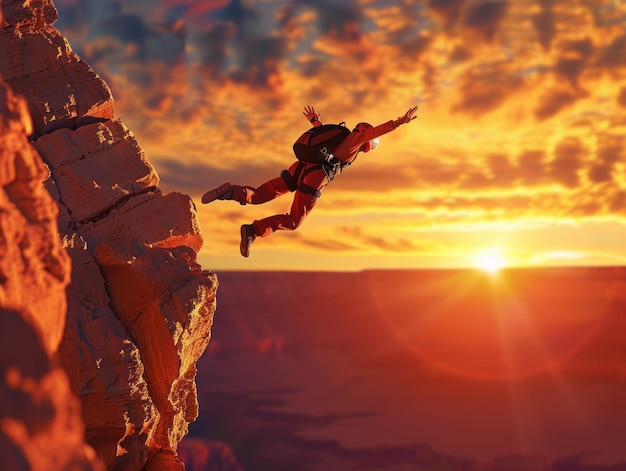This captivating photograph, teetering between realism and artistry, captures a vivid moment during sunset in a desert landscape. Dominating the foreground is a rugged, reddish-yellow rock formation on the left-hand side, from which a man is leaping. The jumper is dressed in an orange jumpsuit, complete with a parachute backpack and helmet, indicating he is base jumping. He is centered in the image, arms extended, just beginning his exhilarating descent. The sky above is a canvas of dramatic clouds interspersed with patches of blue, bathed in the warm, golden-orange hues of the setting sun, which peeks through the horizon, suffusing the entire scene with a stunning glow. The clear day enhances the visibility of every detail, from the rocky terrain to the dynamic sky, creating a strikingly vivid and surreal portrayal of adventure and nature.